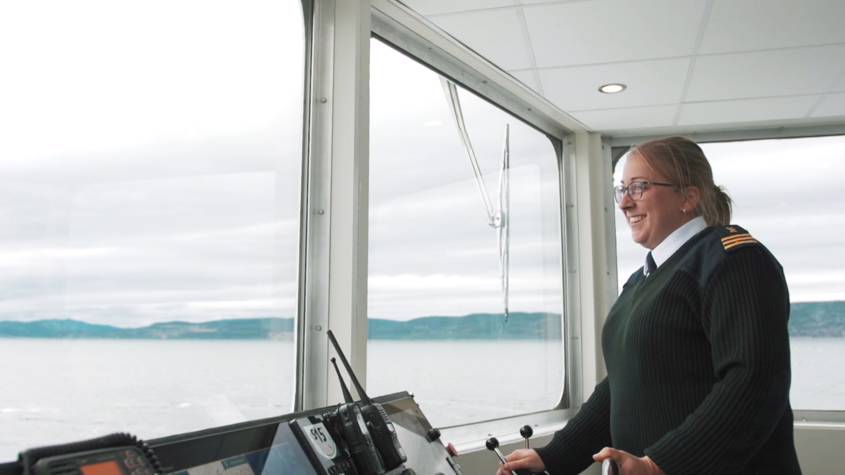In the photo, a woman, who appears to be the captain of a ship, stands in the control room on a misty lake with a mountain range visible through the large front and side windows. The sky and sea share a grayish, foggy hue, adding a serene, almost mystical backdrop. Inside, the control room has a white ceiling with a diamond pattern and a round light. The woman, smiling warmly, is of medium build with darker blonde hair pulled into a ponytail and adorning glasses. She wears a dark green or black long-sleeve sweater with a white collared shirt underneath, a dark tie, and three gold stripes on her shoulder indicating her rank. Her left hand grasps the top of a steering wheel while her right hand holds a lever. The control panel in front of her features a touchscreen pad, assorted equipment, and two radio walkie-talkies. One of the large front windows has a windshield wiper, emphasizing the practical aspects of navigating through such conditions. A white earring in her left ear and her overall composed demeanor suggest both confidence and command, reinforcing her role as the ship's captain.